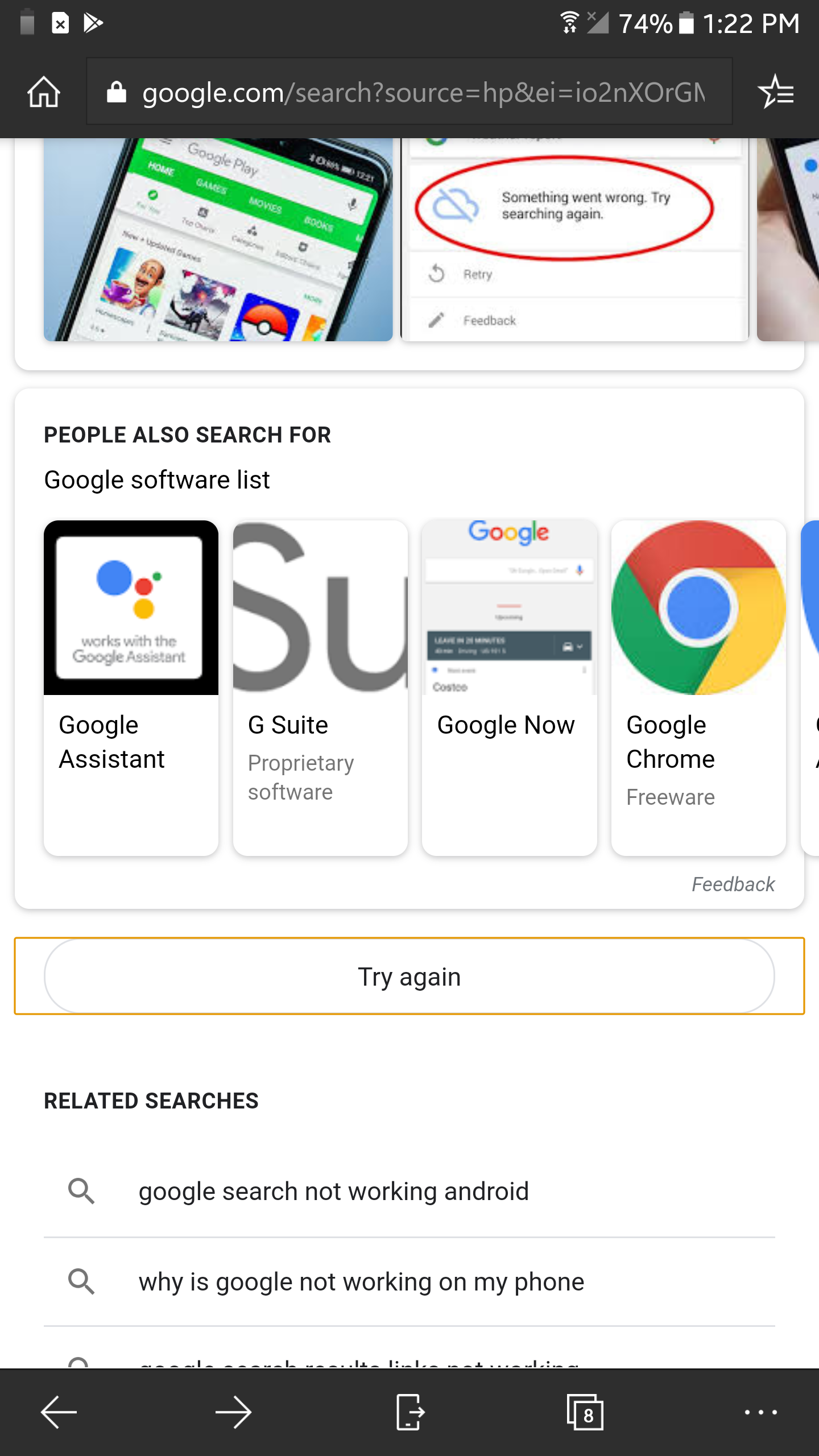This image appears to be a screenshot from a cell phone displaying a web search result page, as indicated by several on-screen elements. The top portion of the screenshot shows a black status bar containing the time, battery level, and Wi-Fi status on the right side, and a small white house icon followed by "google.com" with some additional URL text on the left side.

Below this status bar is the main content of the webpage. On the left, there is a photo of a cell phone displaying what seems to be the app page for a game. On the right side of the image, there is another close-up photo of a cell phone with a large red circle highlighting the message: "Something went wrong, try searching again."

Below these images, there is a section titled "People also search for." This area features several horizontally aligned icons that resemble cell phone screens. The first icon shows colorful dots representing the Google Assistant with the caption "Works with the Google Assistant." The second icon shows the initials "SU" paired with "G Suite." The third icon displays "Google Now." The fourth icon features the Google Chrome logo and is labeled "Google Chrome Freeware."

Further down the page, there is a conspicuous red box around a white square with a yellow border containing the text "Try again." At the bottom of the screenshot, the page lists related search queries, such as "Google search not working Android" and "Why is Google not working on my phone."